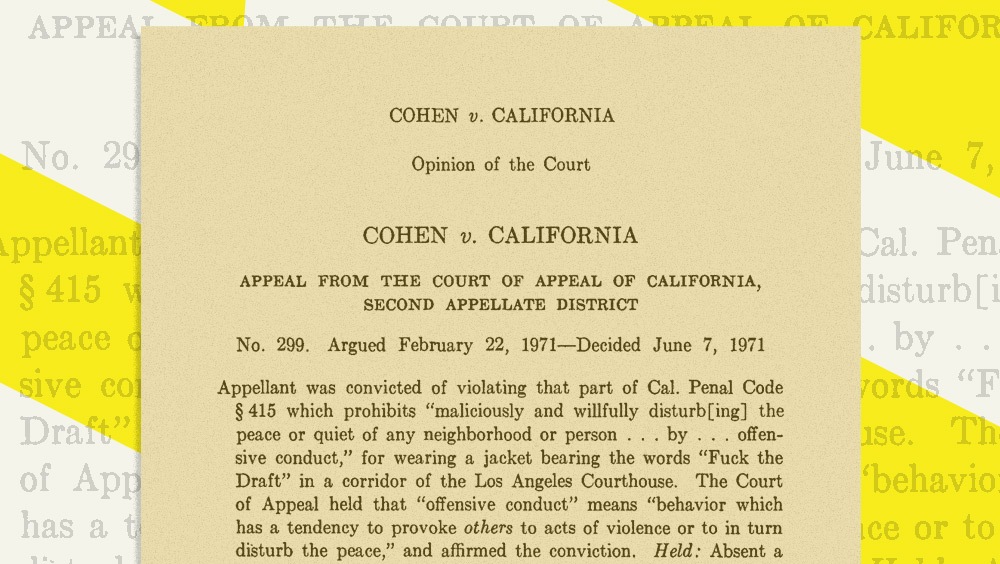This image depicts a legal document central to the scene, specifically a court opinion from the case *Cohen v. California*, decided by the Court of Appeal of California, 2nd Appellate District, on June 7, 1971. The document, printed on tan or light brown paper, addresses the appellant's conviction under the California Penal Code for maliciously and willfully disturbing peace by wearing a jacket bearing the phrase "Fuck the Draft." The background features an enlarged, partial view of the legal text with a white backdrop and yellow stripes. The text itself appears in a dark brown font, emphasizing the judicial style of the document. The appellate court defined offensive conduct as behavior likely to incite violence or disrupt the peace, affirming the conviction.